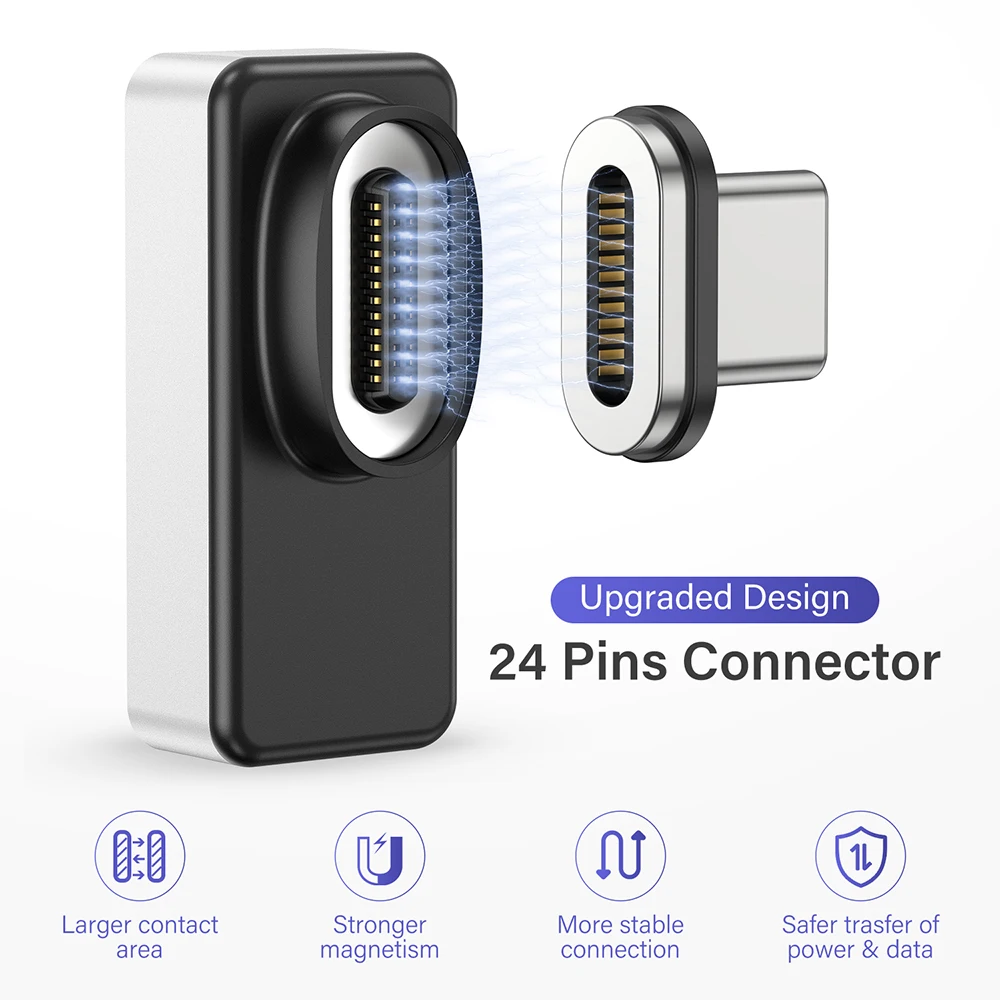The image is an advertisement showcasing an upgraded design 24-pin connector against a white background. Dominating the center are two components of the connector: the left piece resembles a USB Type-A port with an area accommodating a USB Type-C insert, while the right piece, a USB Type-C adapter, is depicted sliding into place. The connector is primarily black with a silver front and features blue accents illustrating magnetism and electrical activity between the two segments. Text on the image reads "upgraded design 24 pins connector," with "upgraded design" highlighted in purple. Below, several symbols accompanied by text—also in purple—promote the product’s features: larger contact area, stronger magnetism, more stable connection, and safer transfer of power and data.